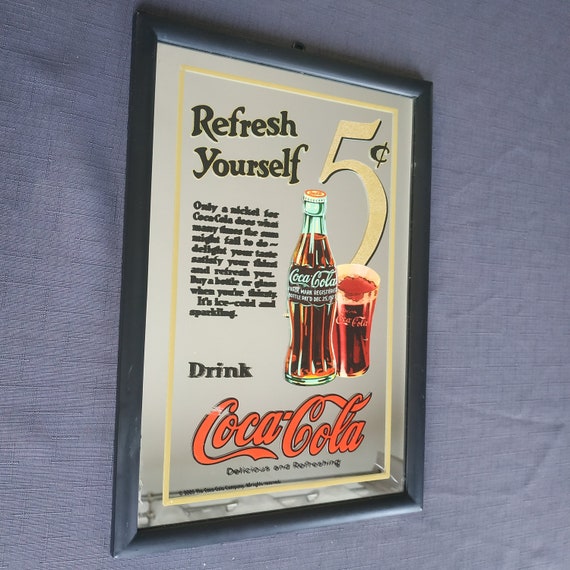Framed against a gray wall, this vintage Coca-Cola advertisement exudes nostalgic charm. The black-framed sign features an inner bevel of light yellow matting, encapsulating a gray background. Prominently, the text "Refresh Yourself" is on the left side in black lettering. Below this, a paragraph describing Coca-Cola appears, though the small text is somewhat blended together. Dominating the right side is a large yellow number "5" with a black cent sign, denoting the beverage's cost of five cents. Beneath the "5," there is an old-fashioned glass bottle of Coca-Cola, showcasing the iconic white script logo, alongside a vintage Coca-Cola glass filled with the effervescent drink, crowned with a frothy head. Further down and to the left, the word "Drink" appears in black, with the classic red Coca-Cola script logo below it. Additional phrases like "Delicious and Refreshing" and "Ice Cold and Appealing" can be made out, reinforcing the advertisement's retro allure.